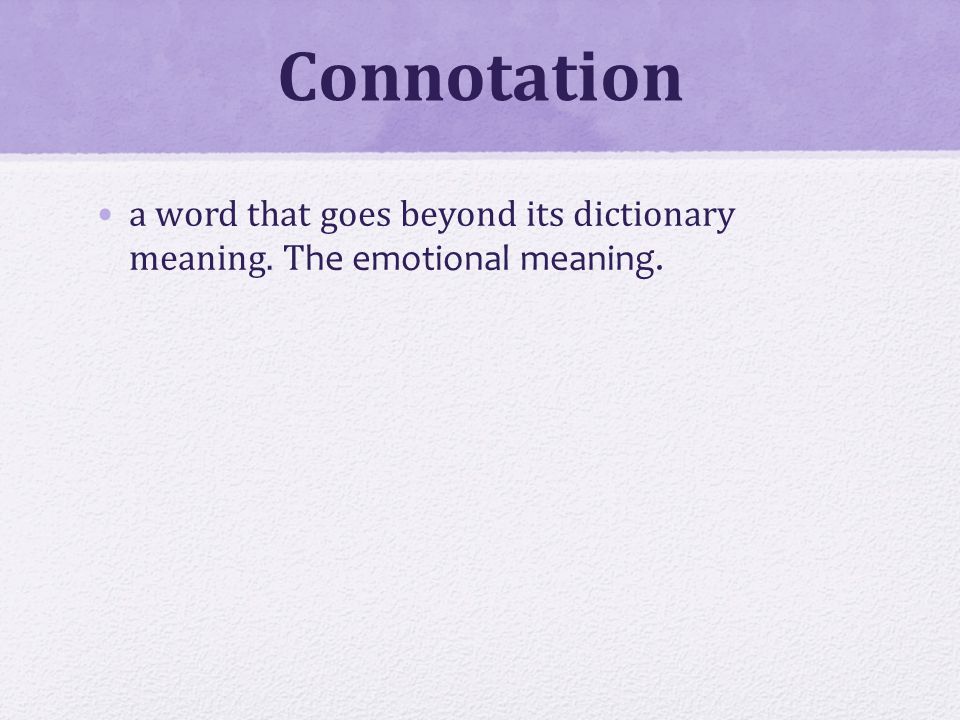The image is a two-toned, rectangular presentation slide or flashcard, predominantly purple, resembling materials used for classroom learning or educational posters. The top section features a darker purple rectangle containing the word "connotation" in bold, large, black font, making it easily visible from a distance. Below this is a larger light purple area with a definition of "connotation," also in a sizable font for legibility. The definition provided reads: "a word that goes beyond its dictionary meaning; the emotional meaning." Notably, this area includes a small bullet point next to the text. Both the darker and lighter purple regions exhibit a textured pattern reminiscent of a sponged paint effect, adding a tactile dimension to the image. The overall layout leaves ample open space in the light purple section, suggesting potential for additional content or expanded explanations.